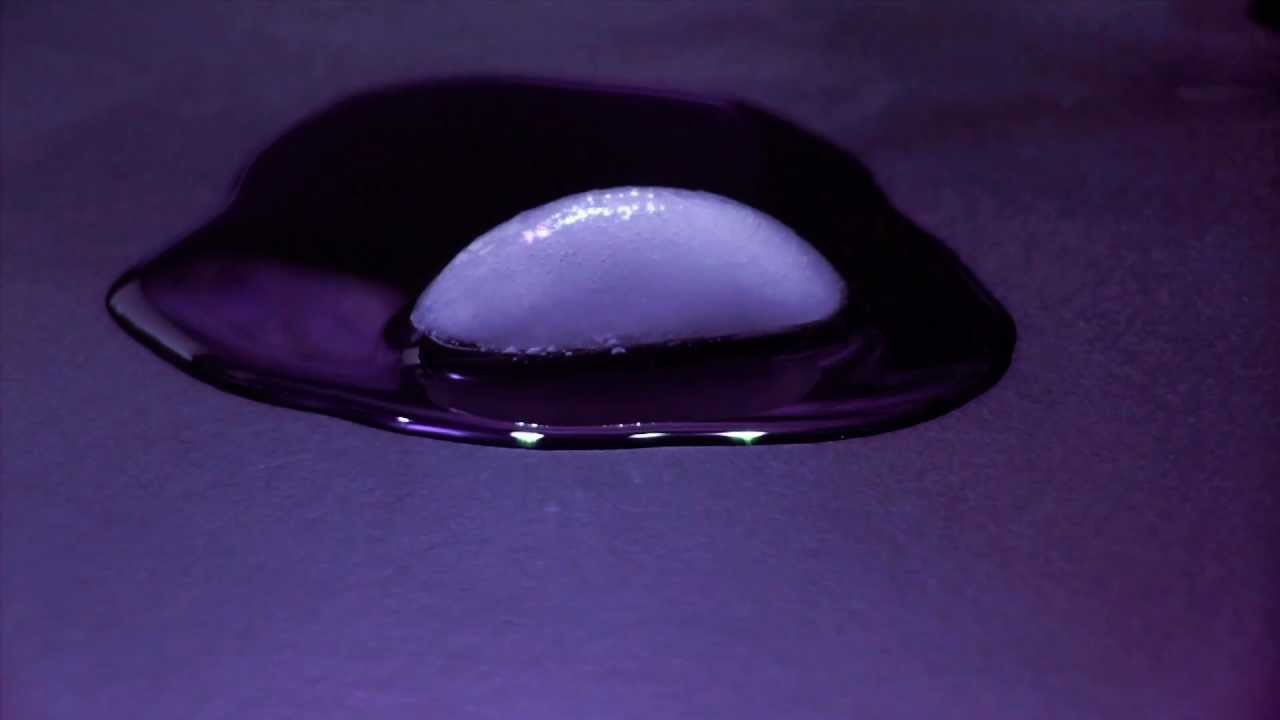The image displays a small, half-melted ice cube with a purple hue, somewhat resembling the shape of a fingernail. The melting ice cube is surrounded by a puddle of water, which reflects light towards the front. The puddle, approximately an inch in diameter, deepens in color due to the dark purple backdrop on which it sits. This background transitions to a lighter shade of purple towards the front and becomes very dark near the top right corner. Small light reflections can be seen both on the ice cube and within the puddle, enhancing the ethereal and captivating visual effect.